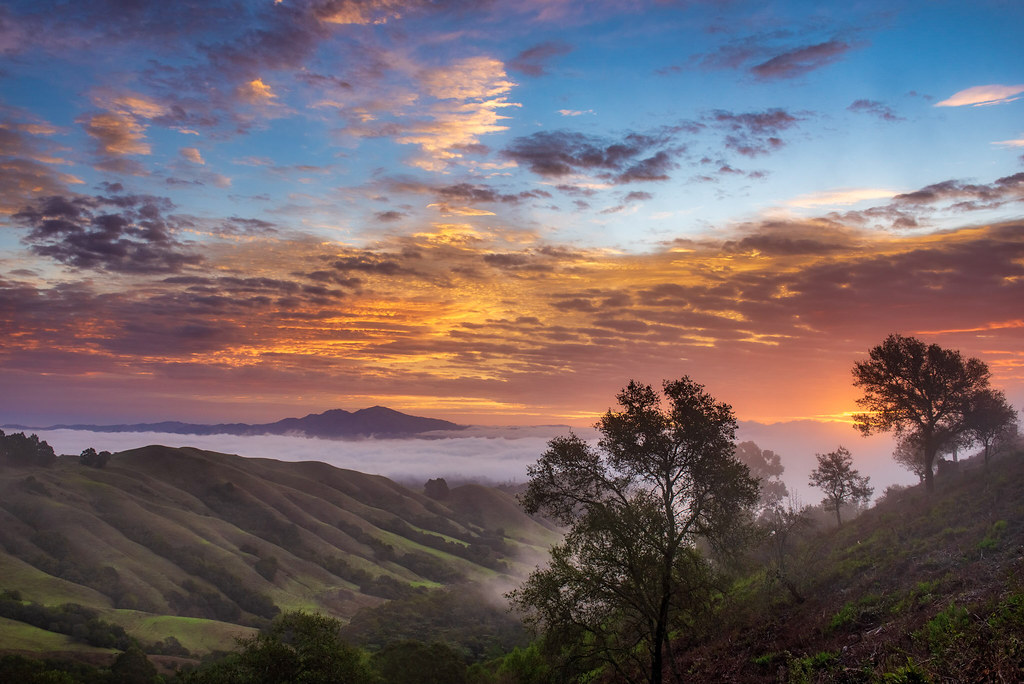The image depicts a breathtaking sunset over rolling green hills and distant mountains. The sky transitions beautifully from a deep blue at the top to vibrant shades of yellow, orange, pink, and dark purple near the horizon, where the sun appears low and almost on fire. The clouds, tinged with orange and yellow hues, add drama to the scene. Below the sky, the landscape features lush greenery; the foreground is dominated by dark green hills dotted with various bushes and trees, while the more distant hills display an array of plant life and trees of different sizes. Off to the right, a closer hill is topped with taller trees and more detailed foliage. In the distance, a mountain peak is visible and veiled in white fog, enhancing the mystical ambiance. The image is completed by the serene presence of light-colored gray water at the valley's base, leading the eye towards a small island on the horizon. Overall, this rich and detailed painting captures the serene and dynamic beauty of nature during a sunset.